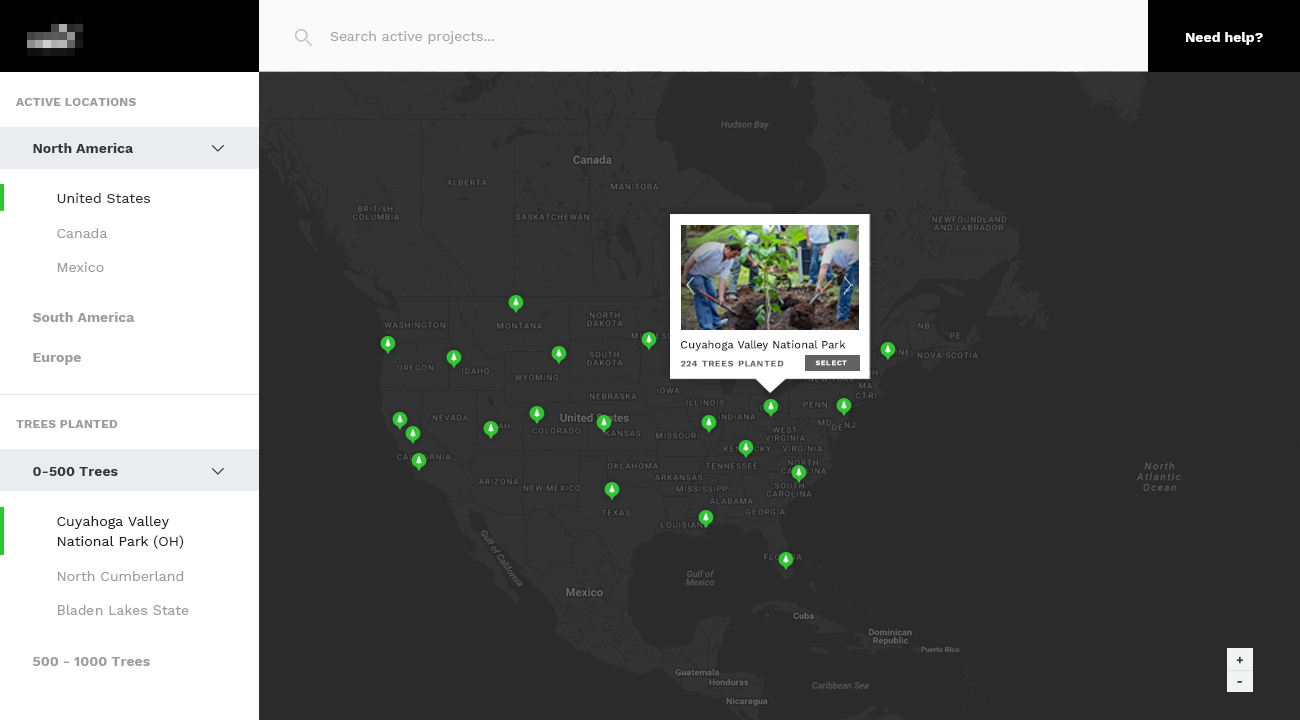The image depicts a dark map with numerous green dots indicating various locations. At the top, there is a search bar labeled "Search Active Projects." On the left side, a panel titled "Active Locations" lists regions such as North America, specifically highlighting the United States. The text mentions "Trees Planted: 0-500" in Chattanooga Valley National Park, Ohio. 

Several green dots across the U.S. suggest multiple active projects in different areas. The map further details a specific project in Chattanooga Valley National Park where 224 trees have been planted. Accompanying the map is a photograph showing volunteers planting large trees in a row, rather than saplings. The volunteers, donning blue jeans and t-shirts, are actively involved in the tree-planting effort.